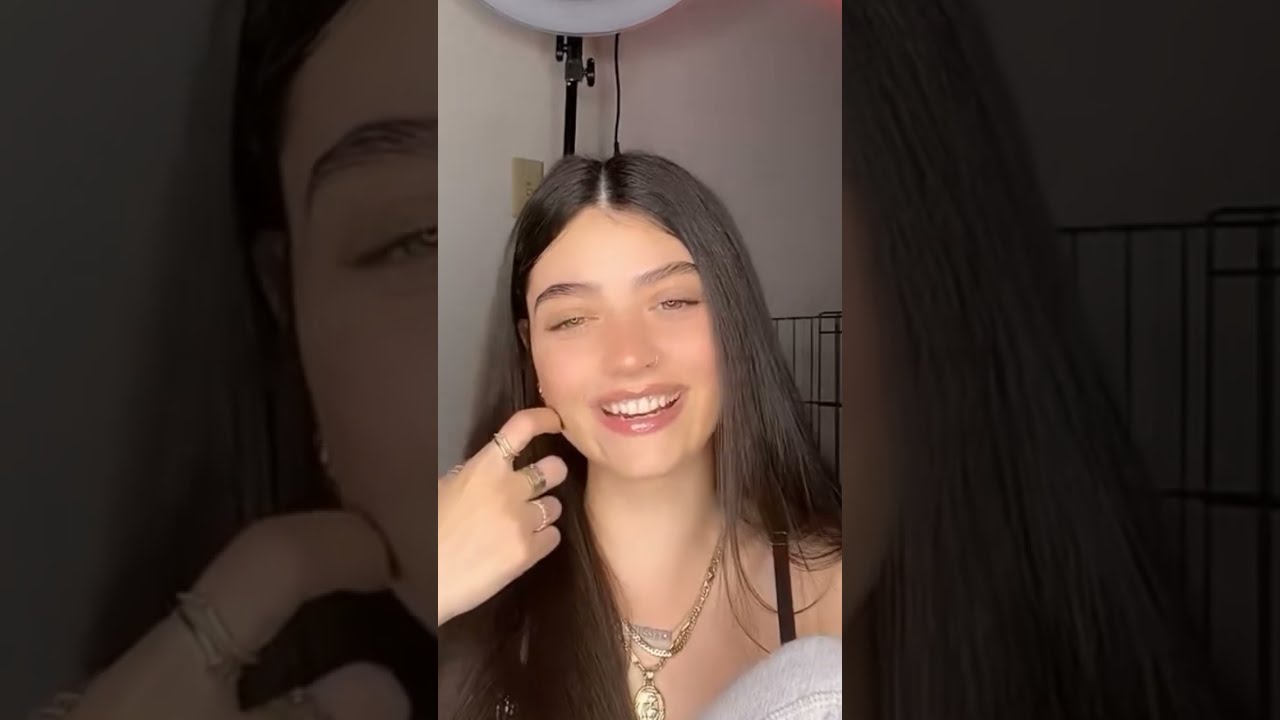In this vibrant, color portrait, a young woman with long, straight dark brown hair smiles warmly at the camera, her glossed lips slightly parted. Her expressive eyes are framed by her sleek hair, and her right hand is raised, her index finger gently touching her cheek. Adorning her fingers are multiple rings, excluding her pinky, adding a touch of elegance to her casual pose. Around her neck, she wears a combination of two or three delicate gold necklaces, though she is also described at times as wearing a silver necklace with a pendant.

The background reveals she is indoors, with white walls and lighting equipment partially visible. A narrow black stand, possibly for lighting, and a slim black frame—perhaps for a piece of furniture or equipment—can be seen. Additionally, a beige wall outlet is noticeable, peeking from behind the left side of her head. Meanwhile, a black strap falls over her shoulder, hinting at her outfit. The overall composition suggests the photo was taken with a cell phone, likely in portrait mode, which has subtly darkened the edges to emphasize her serene expression.